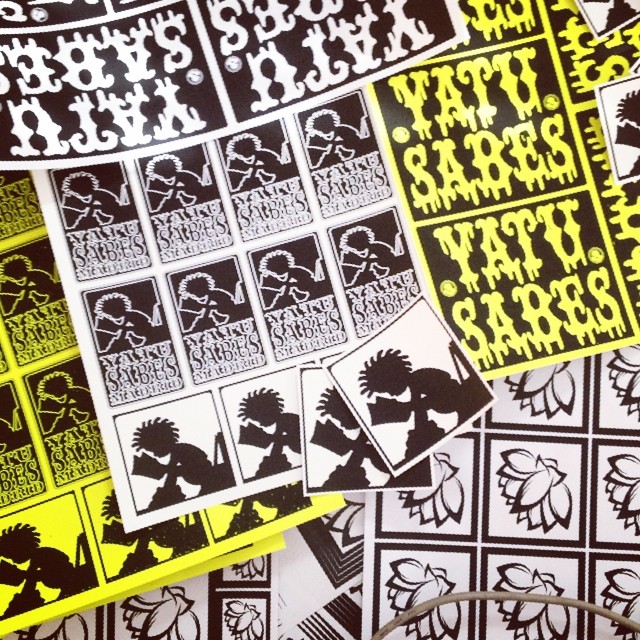The photograph displays an assortment of freshly printed papers stacked haphazardly over one another, featuring a blend of colors primarily in black, white, and yellow. Dominating the center is an image consistently shown across several papers: a black silhouette of a person with scraggly hair, sitting on steps, seemingly engrossed in reading a piece of paper or a newspaper. This image is intricately detailed, revealing large tennis shoes and suggesting a narrative through its portrayal. The text "Yatu Seibus" is prominently repeated across different sheets in both yellow and white against black backgrounds. Some papers also feature small, square patterns showcasing a flower imprint, adding a decorative element to the scene. In the bottom right corner, a piece of grey wire can be distinctly seen, subtly hinting at possible connections between the scattered designs and themes.